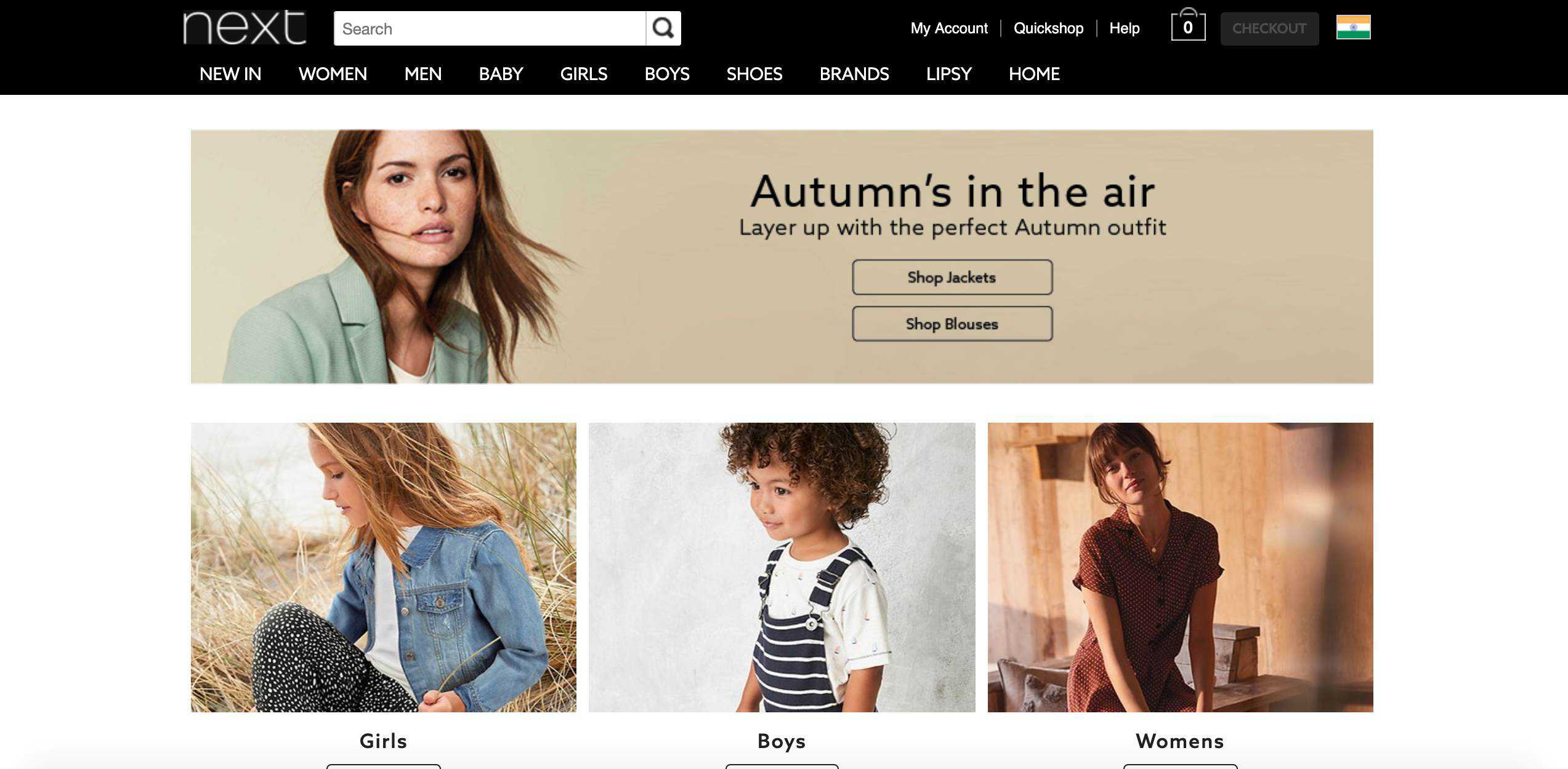This is a detailed screenshot of the NEXT website. The top banner is a deep, dark blue and prominently displays the word "NEXT" in crisp white lettering. To the right of the logo, there's a white search box with the placeholder text "search" inside. Below this banner, a series of selectable tabs are lined up in white letters: "new in," "women," "men," "baby," "girls," "boys," "shoes," "brands," "Lipsy," and "home."

The main section of the website features a clean, white background. At the top, there's a large tan rectangle showcasing a woman's face. To the right of this image, a promotional message reads: "Autumn's in the air. Layer up with the perfect autumn outfit." Below this message, two buttons invite users to "Shop Jackets" and "Shop Blouses."

Below this promotional area, there are three smaller images arranged horizontally. The first image on the left shows a young girl wearing a blue jean jacket. The middle image features a young boy dressed in black and white striped overalls over a white t-shirt. The third image on the right highlights the women's section, depicting a woman in a dark red blouse.